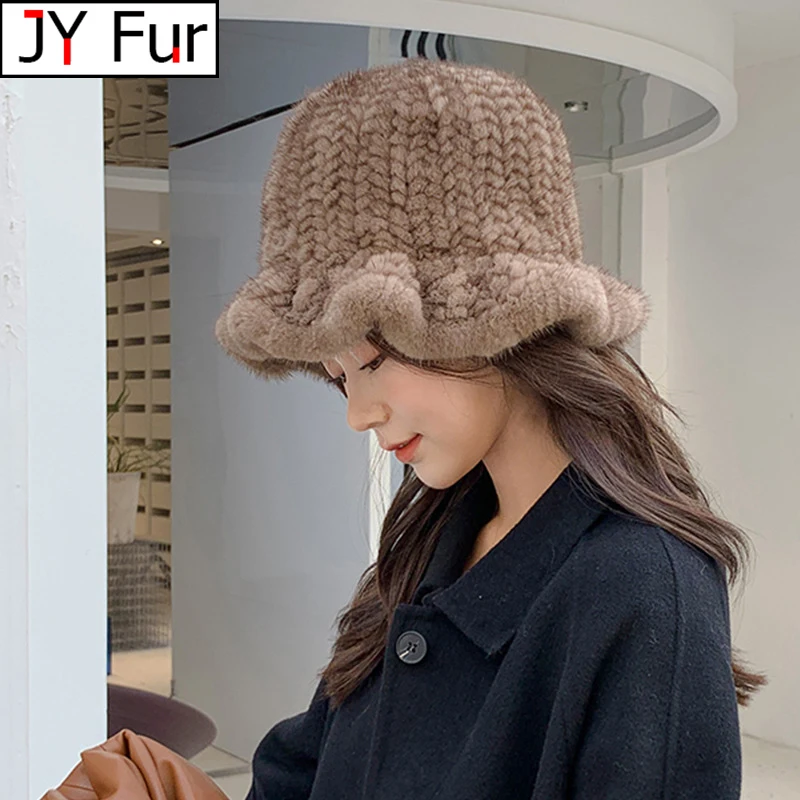The image depicts a photorealistic mannequin of a young Asian woman with extremely pale skin and long brown hair, suggesting she is of Japanese descent. She is dressed in a black peacoat with a golden button on the collar, and a fuzzy knitted light gray-beige cap with a wavy brim. The mannequin is facing left, with her gaze directed downwards, and seems to be holding or looking at a brown leather item at the bottom of the image, possibly a purse. The background reveals a shopping mall setting with white and gray walls, white pots with plants, and a store entrance. In the upper left corner of the photo, a white rectangular sign with a black border reads "J-Y Fur" in black and red text.